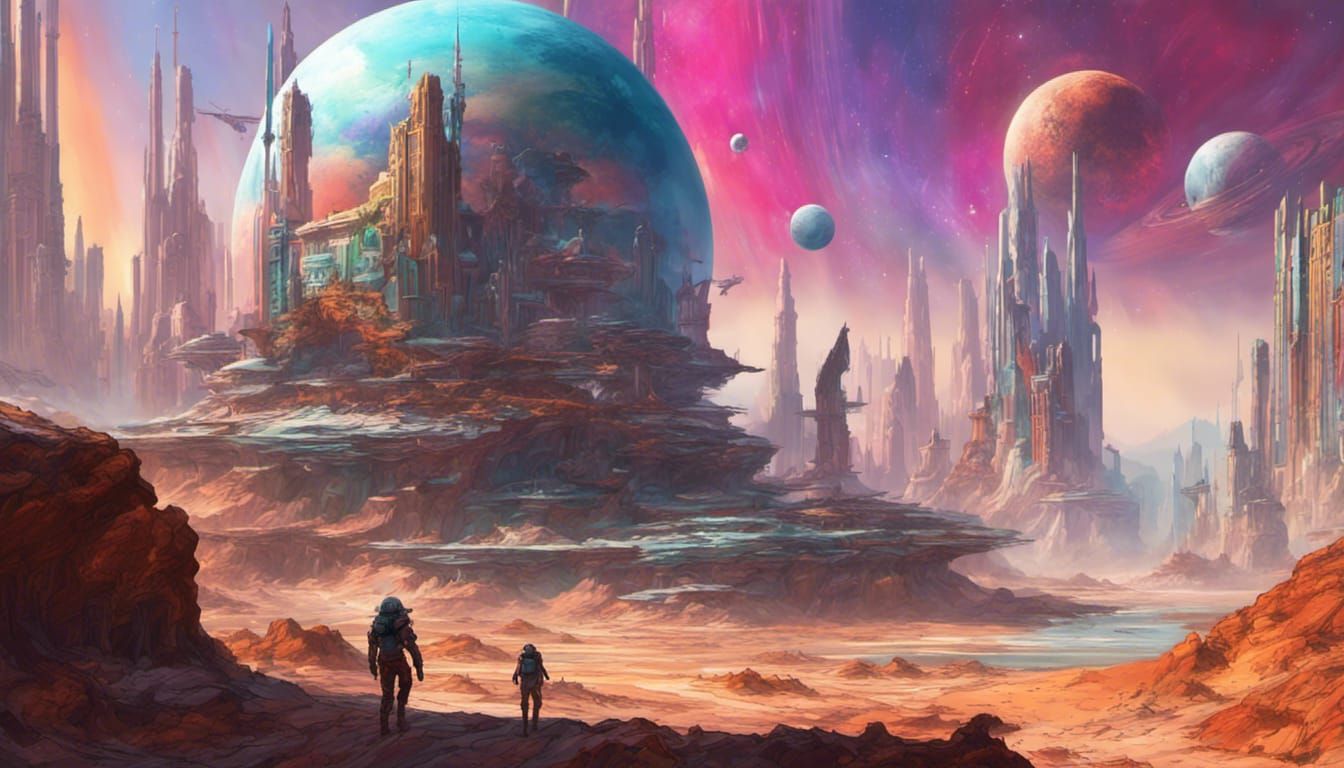This digitally created, multi-color fantasy scene depicts a barren alien landscape with intricate details. A pair of astronauts, cast in shadow, venture across the brown, arid ground toward a towering rock formation crowned with an elaborate building. The terrain, mostly devoid of vegetation, subtly transitions to what appears to be water on the right. The sky bursts with a spectrum of colors—yellow, orange, blue, purple, pink—creating an ethereal backdrop. Dominating the scene is a massive planet behind the rock structure, with a cluster of four smaller planets scattered across the upper expanse. The futuristic cityscape boasts tall buildings and spires, seamlessly integrated with rock layers and interspersed with trees. The artistry meticulously blends elements to convey the essence of a distant, otherworldly environment.